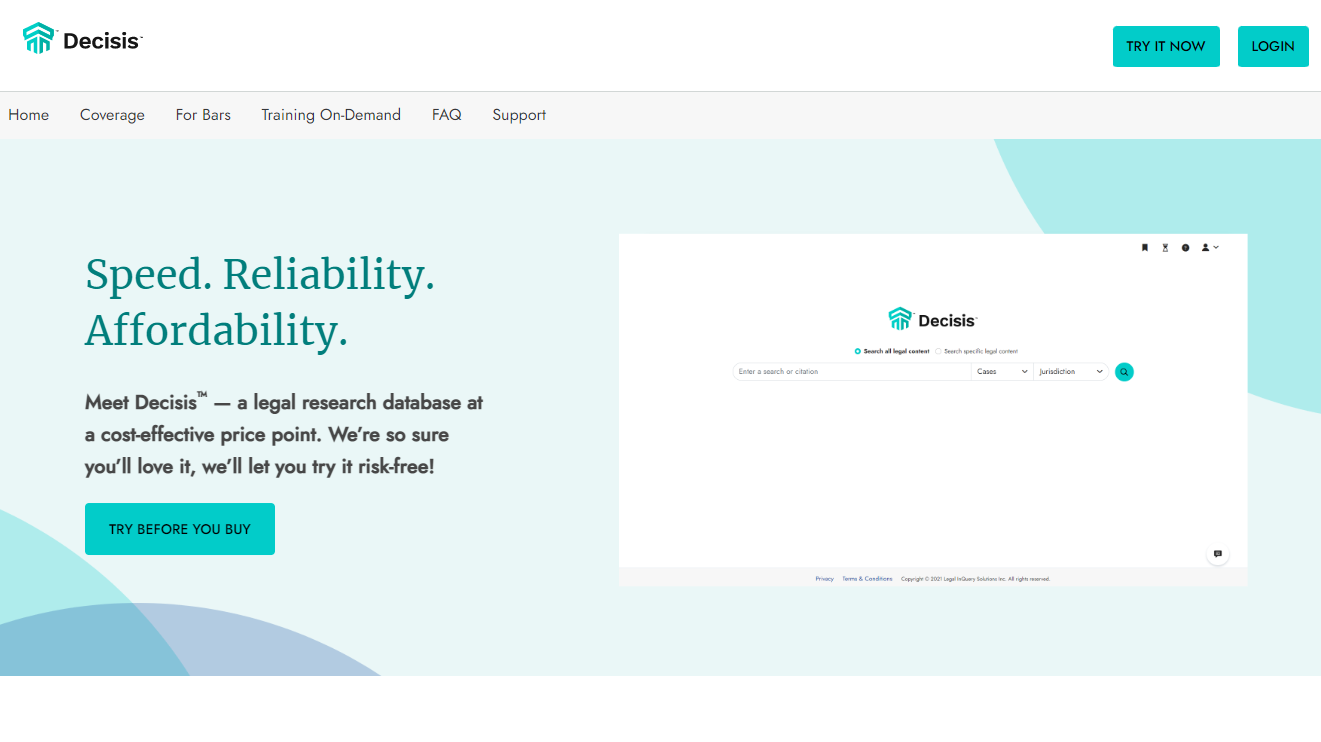This image is a screenshot of the homepage of the Decisys website displayed on a computer screen. In the top left corner, the brand's logo and name, "Decisys," are prominently featured. On the top right, there are two buttons labeled "Try It Now" and "Log In."

The website's color scheme is a harmonious blend of aqua turquoise blues, whites, and other shades of blue. A horizontal menu bar spans the top of the page presenting options like "Home," "Coverage," "For Bars," "Training on Demand," "FAQ," and "Support." 

On the left side of the homepage, a headline and accompanying description are displayed. The headline reads "Speed, Reliability, Affordability," and the description follows with "Meet Decisys, a legal research database at a cost-effective price point. We're so sure you'll love it, we'll let you try it risk-free." Below this text, a blue button reads "Try Before You Buy."

To the right of the descriptive text, there is an image depicting a mock-up of the Decisys platform interface. It resembles a standard search bar page but substitutes the Google logo with "Decisys." There are white fields below the Decisys logo designated for entering search terms and locations, offering a glimpse into the user interface of the Decisys platform for potential customers.